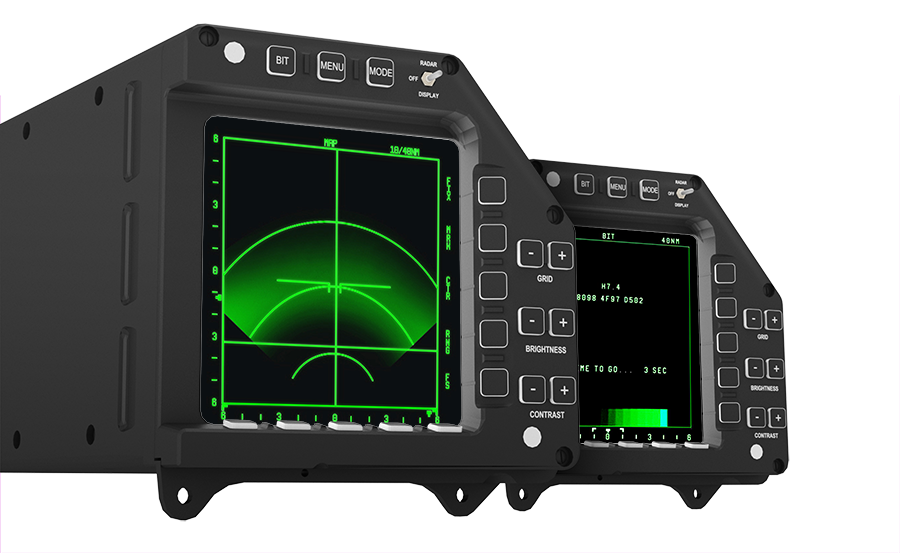The image features two large, boxy machines, both in a dark gray or graphite color, displaying an array of controls and screens indicative of radar equipment. The prominent machine at the forefront has a central square display with a black background, illuminated by bright green lines, numbers, and arches that form a grid-like radar interface. At the top of this machine, there are several control buttons: a white one, and three square buttons labeled "BIT," "MENU," and "MODE," all set against a black background with silver borders. To the right of these buttons is a lever with three positions labeled "RADAR," "OFF," and "DISPLAY."

Below the main display, the front panel hosts additional control features. There are five unmarked black buttons with silver borders, followed by a series of plus and minus buttons for adjusting settings like "GRID," "BRIGHTNESS," and "CONTRAST." The lower portion includes white-circled details that might suggest wheels or structural attachments.

Partially visible in the background is a second, similar machine, mirroring the design and functional elements of the primary one, enhancing the impression of a sophisticated radar system workspace.